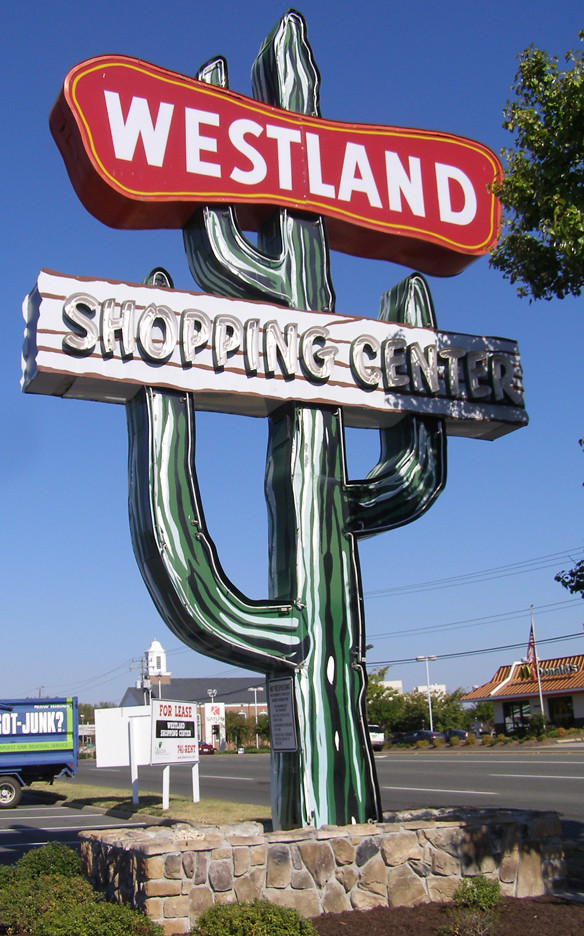A vibrant mid-day scene at Westland Shopping Center is captured with a beautifully clear, cloudless blue sky. In the image, a visually striking sign stands prominently in the foreground. The sign is stylized as a tall green cactus with a sturdy stone base, featuring arms extending from both sides. On the right side, a single arm emerges, while the left side has two arms, all of which support the signage. At the top of the cactus, a red rectangular block with bold white text reads "Westland." Below it, a longer gray rectangle states "Shopping Center," both signs seamlessly integrated into the cactus structure.

To the right of the image, a hint of a McDonald's can be seen, indicating the variety of commercial offerings within the vicinity. On the left side, several "For Sale" signs dot the landscape, suggesting availability of property. In the upper right corner, the lush green leaves of a deciduous tree add a touch of natural beauty to the bustling commercial setting. This detailed depiction effectively combines elements of nature, commercial signage, and surrounding businesses, portraying Westland Shopping Center as a vibrant hub in the community.